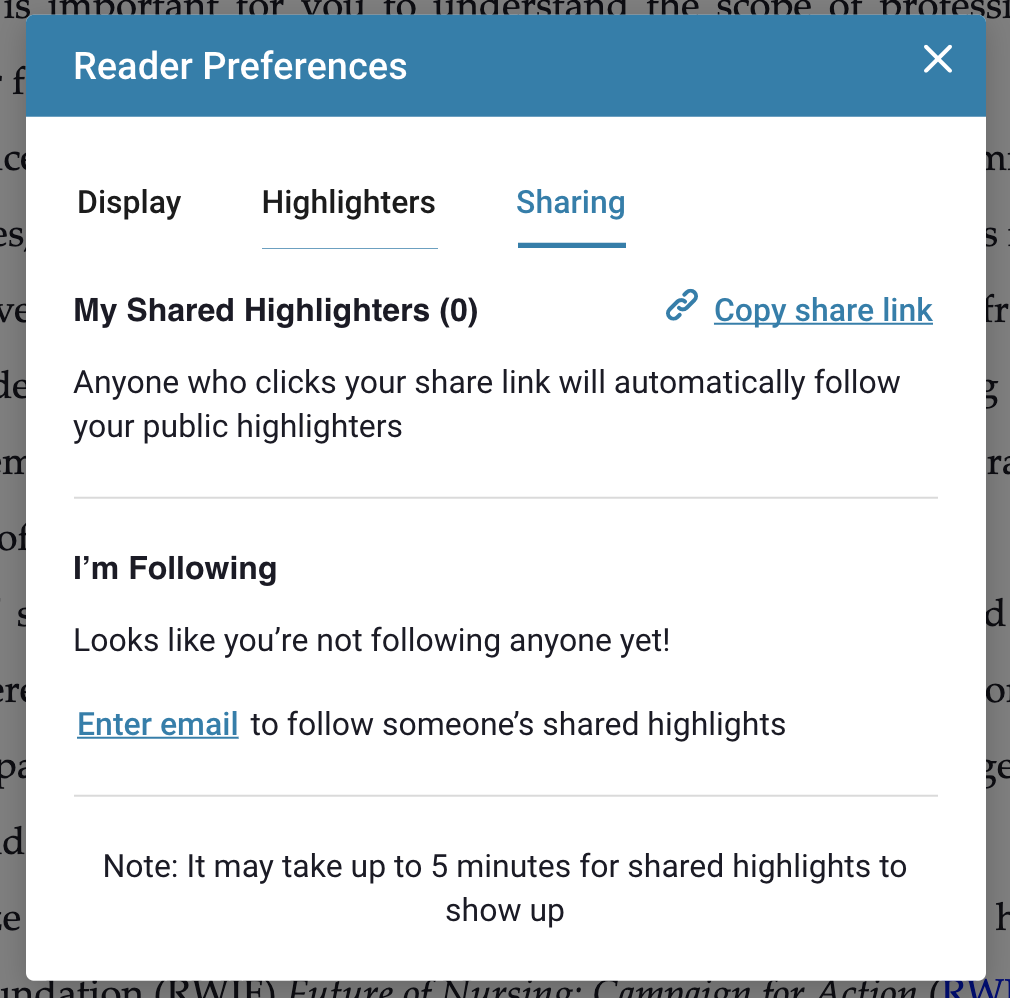Screenshot from an academic readability website displaying user settings under the "Reader Preferences" section. The user is exploring various options to customize their reading experience. The "Sharing" subheading is prominently selected, and the user is focusing on the "Copy this share link" feature. The settings indicate that the user has not shared any highlights yet but has the option to generate shared highlights. Additionally, the interface shows that the user is not currently following anyone but can invite others via email. A notice is visible, informing the user that shared highlights may take up to five minutes to appear, which the user acknowledges.